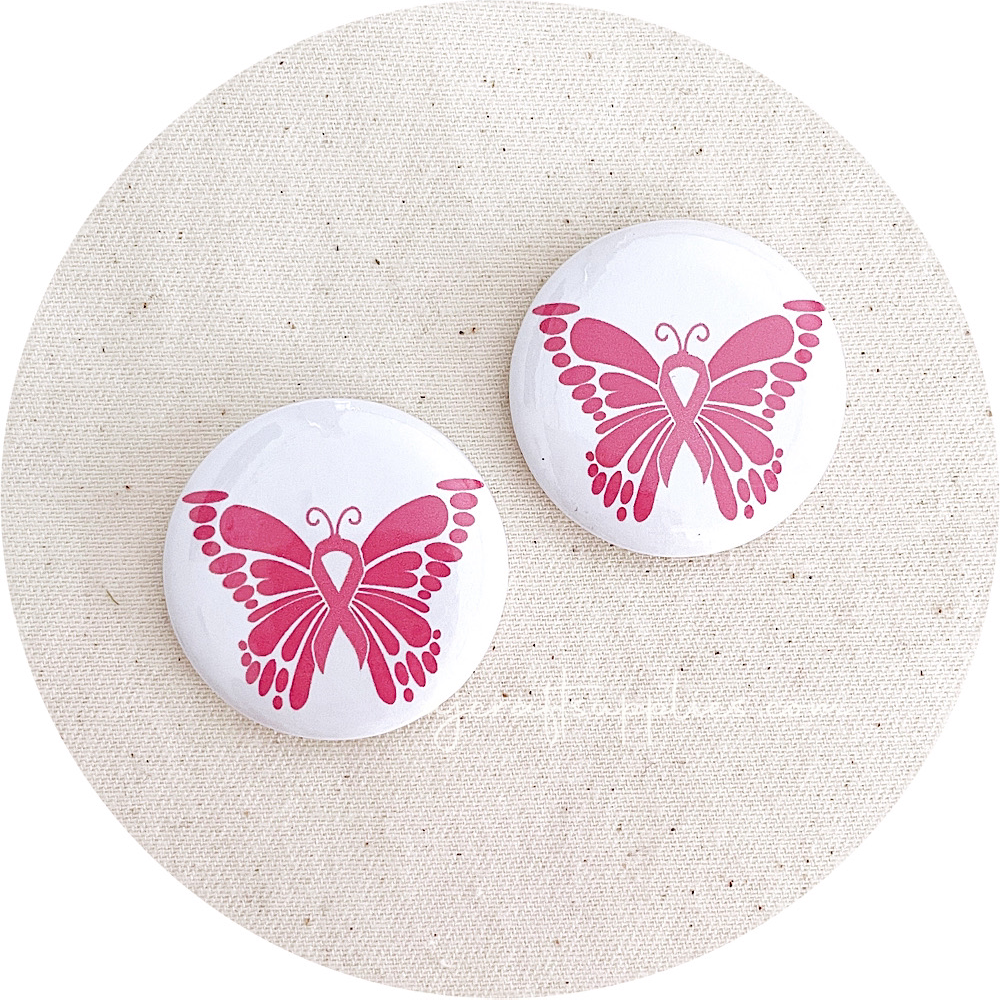This color photograph features two identical round buttons or pins, prominently displayed on a cream-colored, tightly woven, textured fabric background. Each button is white and features a red butterfly design. The butterfly's body forms an awareness ribbon, known for its association with cancer awareness, folded into an X with a curved top and extending into the butterfly's antennae. On the fabric just beneath the buttons, there is barely legible white text, with the readable portion suggesting it might be a website, with the fragment "supplies.com."